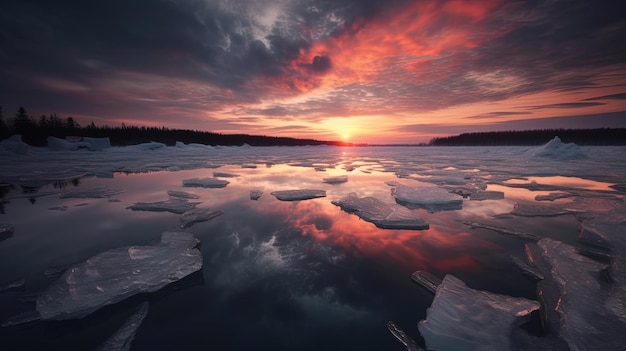This captivating image depicts a serene arctic sunset over a partially thawed glacier lake. The dusky sky is an enchanting mix of purples and oranges, reflecting mesmerizingly on the water's surface. This reflection is interrupted by opaque ice fragments floating on the lake, having broken off from the larger glacier masses encircling the body of water. The horizon line splits the image into two almost equal halves, with the serene lake below and the dynamic sky above.

In the background, the silhouettes of pine trees stretch toward the horizon on the left side of the image, while the right side remains devoid of trees but continues with the horizon's extension. The solid ice formations are more prominent towards the background. The scene is cloud-covered, adding depth and dimension through light play as the sun sets, casting an array of pinks and purples over the landscape. Among the ice piles on the extreme sides of the image, a potential man-made structure, possibly an igloo or a small house, is faintly discernible on the left. This striking image captures the stark beauty and calm of an untouched, natural arctic environment, devoid of signs of life and human activity.